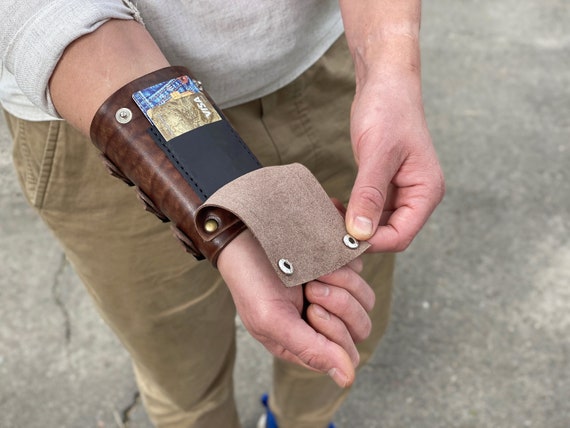The image depicts a detailed close-up of a man standing on a cracked asphalt surface, showcasing a unique wrist accessory on his right arm. He is wearing khaki pants, sneakers, and a light-colored shirt rolled up just below the elbows. His outfit is casual, highlighted by well-trimmed nails and a single visible blue shoe. The focal point is a leather wristlet or bracer, resembling those seen in fantasy settings like Dungeons and Dragons, complete with metal buttons and possibly buckles for adjustment. This wristlet is secured with snaps and unfolds to reveal a hidden compartment designed to hold credit cards. The man is using his left hand to pull down the flap, displaying two credit cards—one blue and another resembling a yellow marble Visa. The wristlet provides a discreet and innovative storage solution, eliminating the need for a traditional wallet. The background and lighting suggest the scene is outdoors on a sunny day.